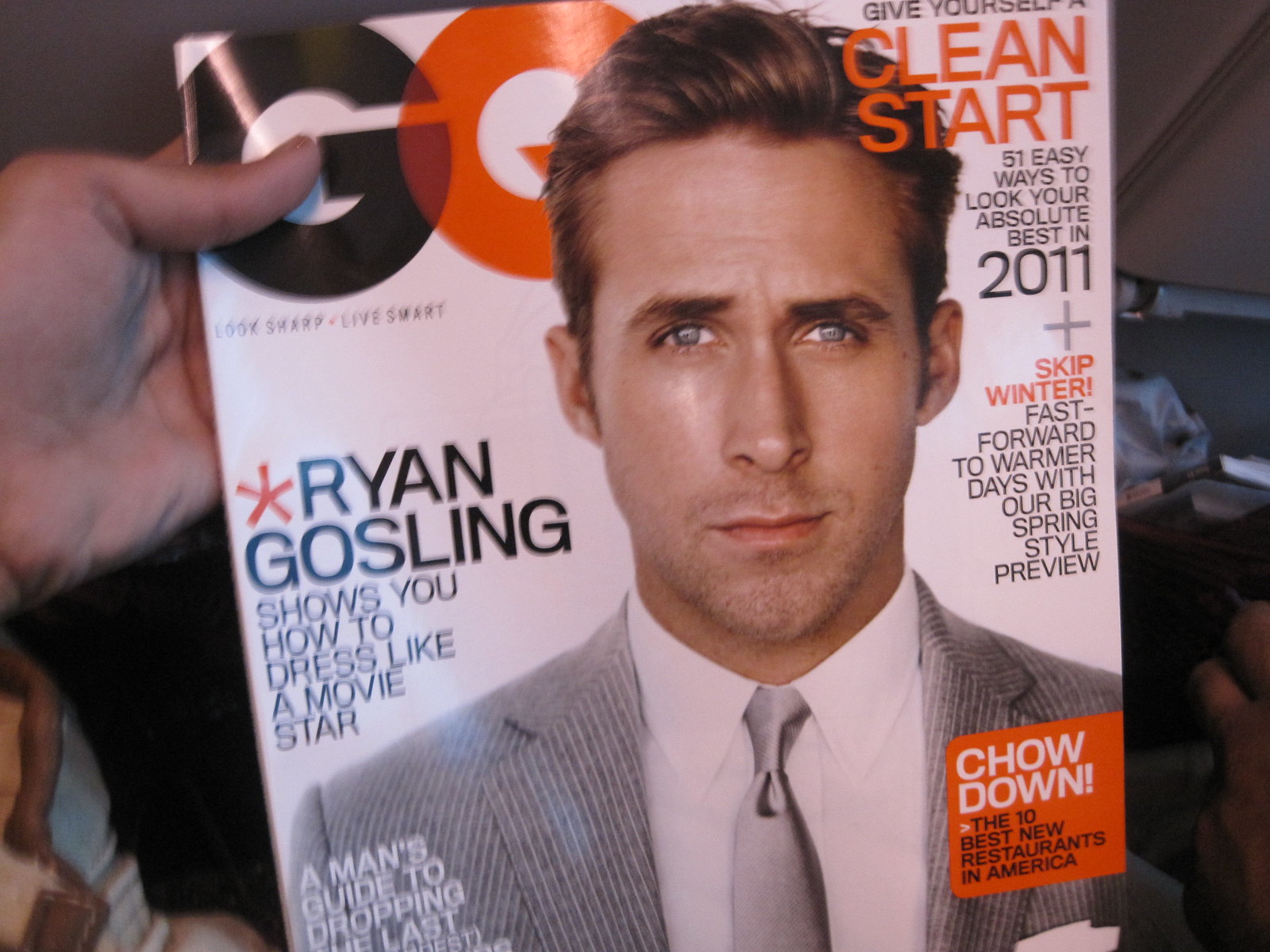**Magazine Cover Description:**

The cover is from the fashion and lifestyle magazine GQ, prominently displayed at the top with its bold logo. The central image features a distinguished person whose identity is not specified. Across the right side of the cover, several headlines appear: "Give Yourself a Clean Start: 51 Easy Ways to Look Your Absolute Best in 2011," followed by "Skip Winter. Fast Forward to Warmer Days with Big Spring Style Preview." In the bottom right corner, there's a small orange square with the words "Chow Down: The Best New Restaurants in America." 

On the left side of the cover, a hand is seen holding the magazine. Below this hand, around the middle, a headline reads "Ryan Gosling Shows You How to Dress Like a Movie Star." Further down, somewhat obscured text partially states, "A Man's Guide to Dropping," with the rest of the line cut off and unreadable. The design is clean and modern, with varied typography enhancing the appeal of each highlighted topic.